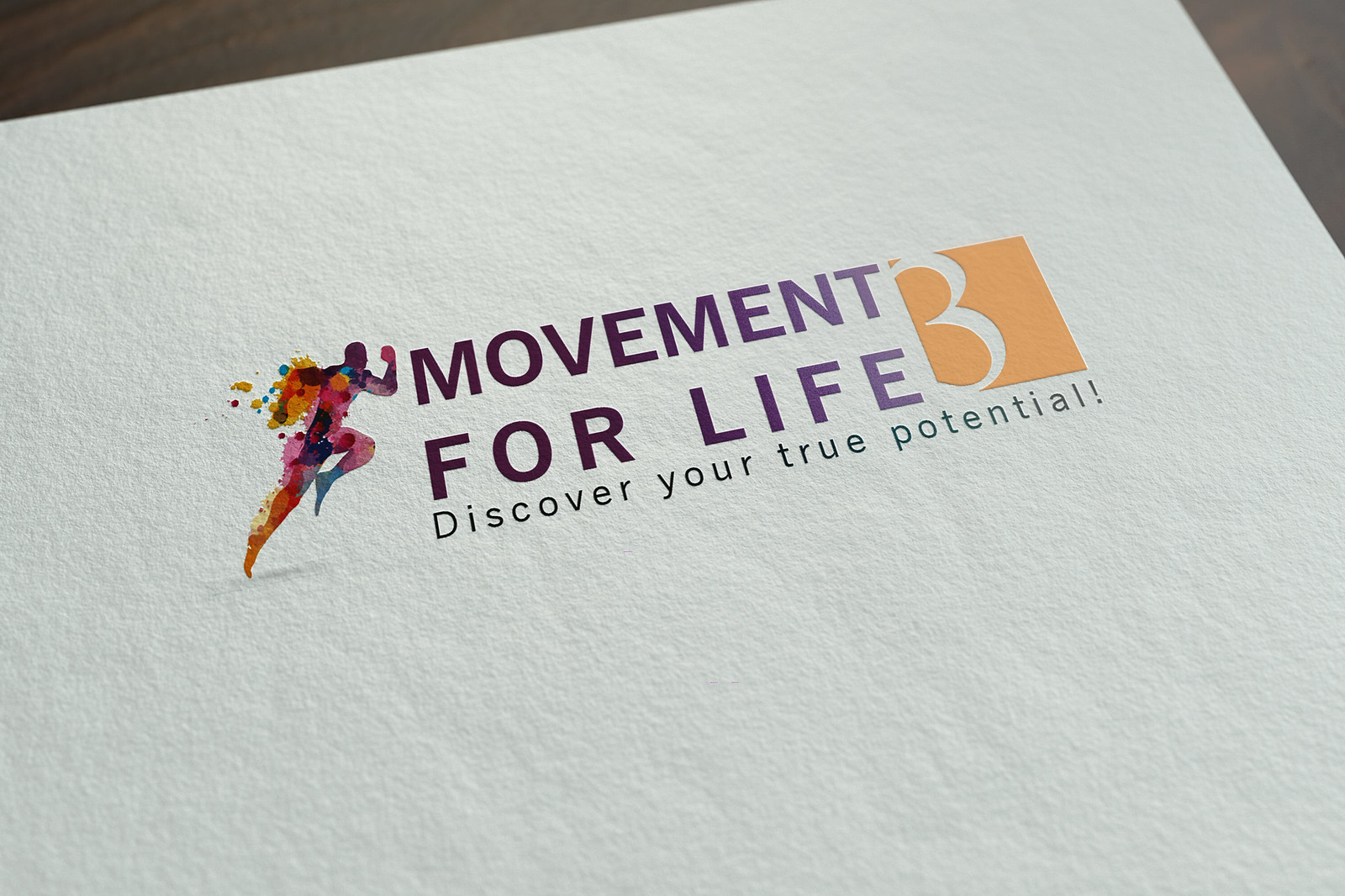The photograph showcases a thick, white business card with a bumpy texture, placed at a slight angle on a dark brown wooden surface that highlights its rich wood grain. The centerpiece of the card is a vibrant, stylized logo of a man running to the right, made up of various colored paint splashes including blue, purple, red, and orange, with his bottom leg in an intense orange shade touching the ground and his arms energetically pumped. To the right of this vivid illustration, the card reads "Movement for Life" in black text across two lines, transitioning into an orange square featuring a stenciled-out number three that reveals the white paper beneath. Finally, the slogan "Discover Your True Potential!" is printed at the bottom in black, adding a compelling call to action.